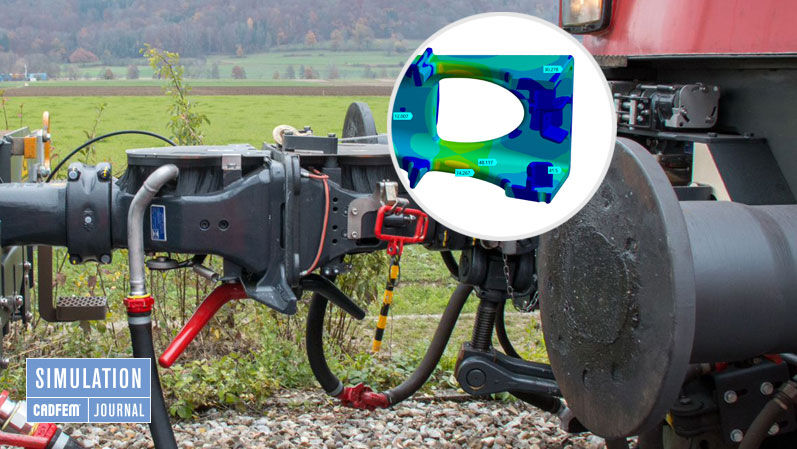This detailed image captures a close-up view of a heavy-duty train coupler, the mechanical device that locks two train cars together. The coupler parts, rendered in heavy gray and dark gray, exude an industrial weightiness. Surrounding it, the ground is covered with rocks, and patches of green grass and bushes stretch towards the background, culminating in distant trees and a cloudy, overcast sky. In the upper right corner of the image, there's an inset that displays a detailed computer analysis model of the coupler components. This inset, part of the "Simulation CADFEM Journal," highlights various parts with multi-colored 3D renderings, including shades of blue and green, and incorporates labels for different components. This inset underscores the use of Computer-Aided Design (CAD) and Finite Element Modeling (FEM) in analyzing the train coupler’s performance and structure.